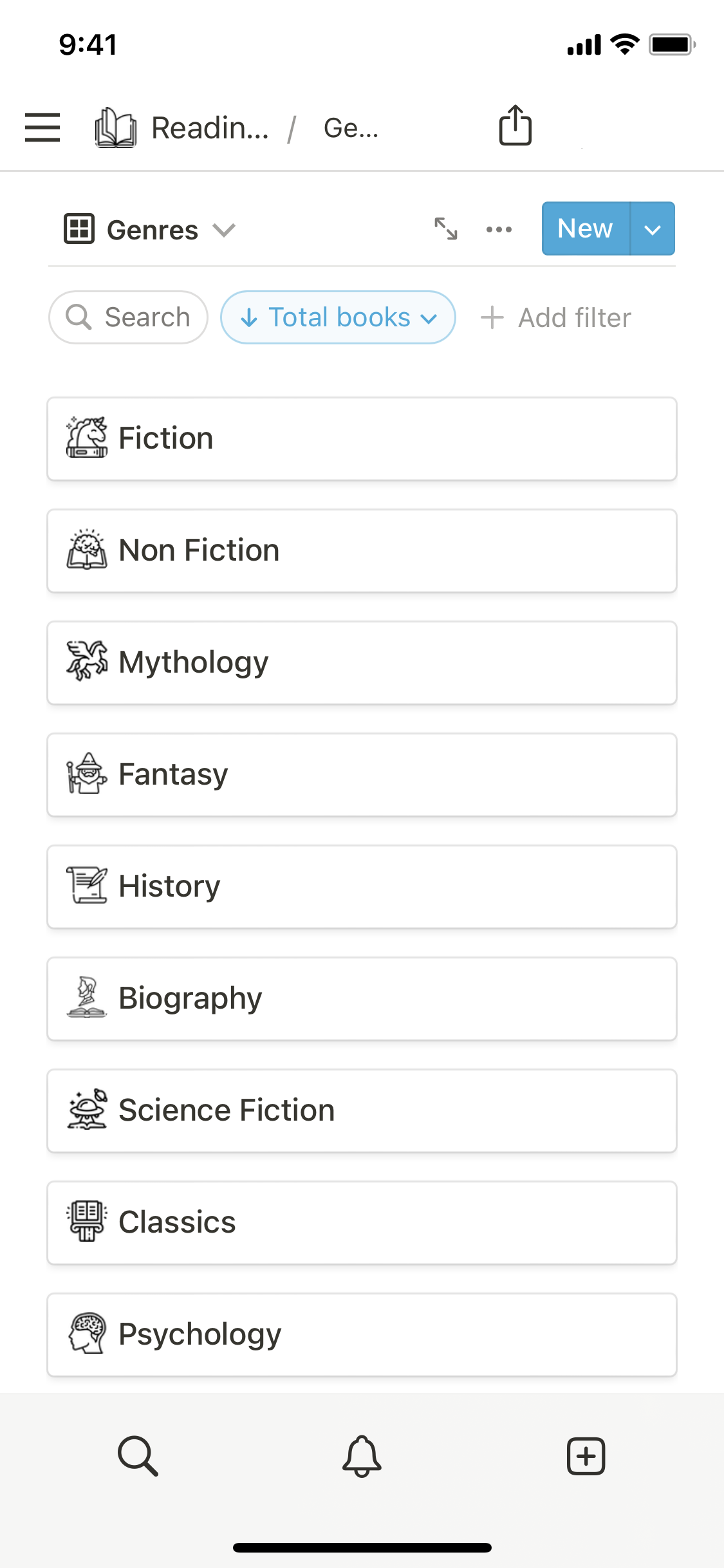Screenshot of a phone showing a reading app interface at 9:41 PM. The phone has nearly a full battery and four bars of reception. Below the status bar, the app displays an image of a hamburger icon and an open book, indicating the current activity is related to reading. The book's title includes the word "Reading GE," and there are options to either go back or download it.

Further down, the screen displays the word "Genres" with a dropdown menu. Next to it is a blue button labeled "New" in white text. Below that, there's a small search bar. Another section titled "Total Books" has an expandable arrow, and there's also an option to add a filter.

The genres listed are as follows: 
1. Fiction
2. Nonfiction
3. Mythology
4. Fantasy
5. History
6. Biography
7. Science Fiction
8. Classics
9. Psychology 

The user can click on any of these genres to select a book to read or have read to them. The person in the image appears to be browsing through these options to find a book to read.